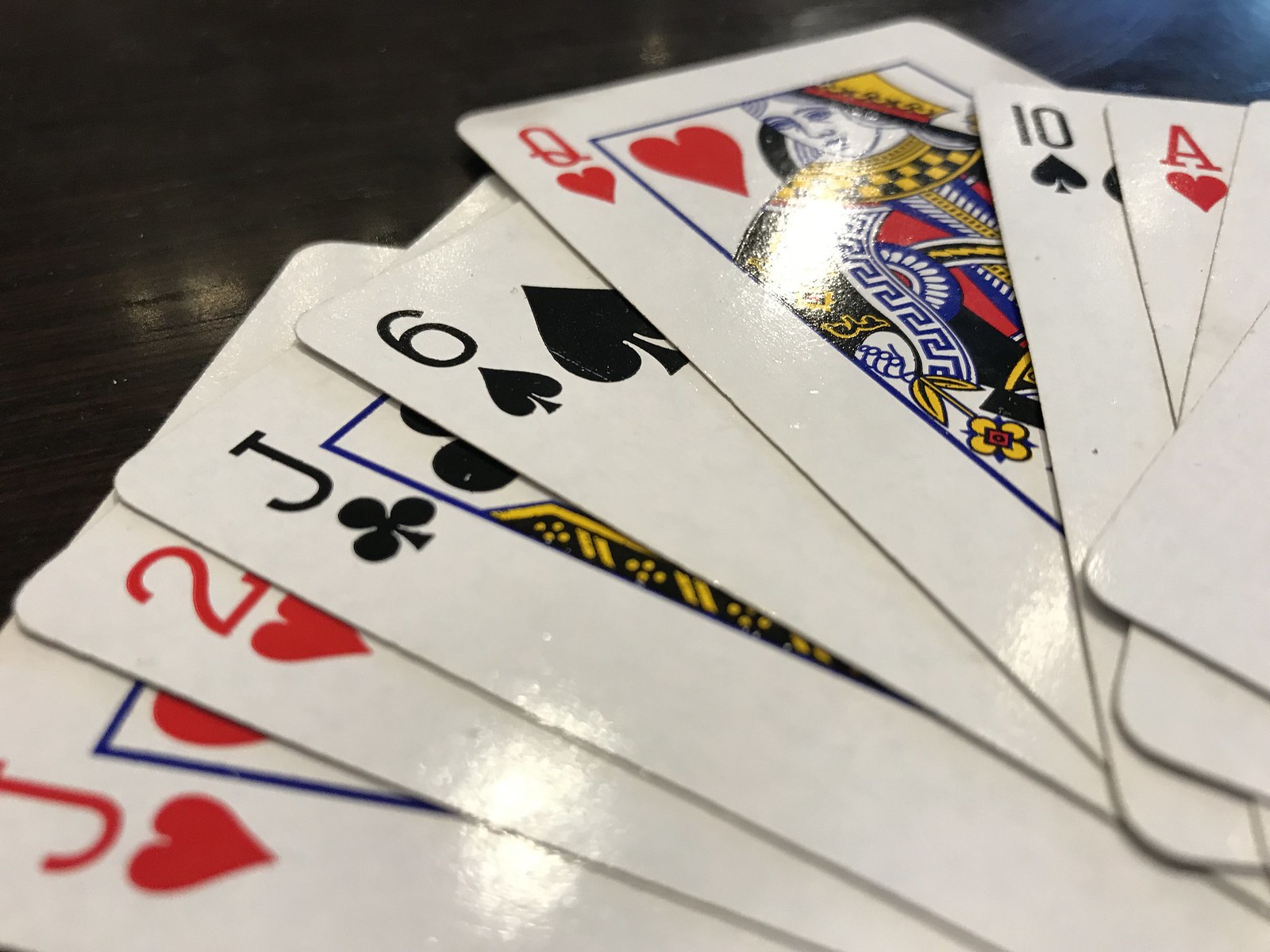A close-up photograph features a deck of playing cards fanned out on a varnished dark wood surface, capturing the intricate texture and reflective qualities of both the cards and the wood. The cards are slightly overlapping, characteristic of how one might hold them in a hand. The visible cards include the Jack of Hearts, Two of Hearts, Jack of Clubs, Six of Spades, Queen of Hearts, Ten of Hearts, and Ace of Hearts, with only the bottoms of a few other cards peeking out. The cards show signs of wear with multiple small dings reflecting light in such a way that it creates bright spots reminiscent of scratches made by a coin, particularly noticeable on the Queen of Hearts. Additional reflective patches of light spread across the Jack of Hearts, Two of Hearts, and Jack of Clubs, adding a dynamic sense of depth to the image.